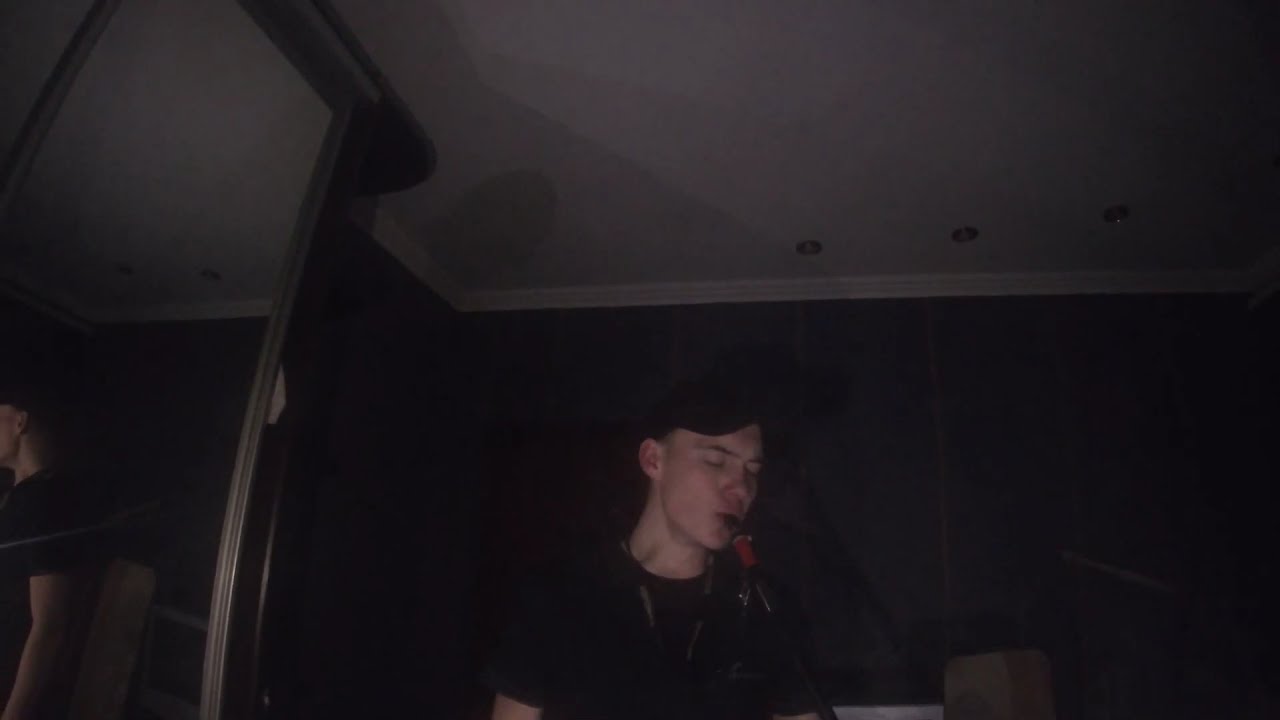The image depicts a young white man in his 20s playing a black saxophone in a dimly lit basement or room with dark walls and a light-colored ceiling. He is positioned at the bottom center of the frame and appears from the chest up. He is wearing a black baseball cap and a black t-shirt and has his eyes closed in concentration. There is a black mouthpiece in his mouth and a neck strap supporting the instrument. To the left of him, a mirror on the wall reflects part of his back, confirming the dark and somewhat grainy quality of the photograph. The room only has dim lighting, enough to faintly illuminate his figure and the surroundings, which include a wooden structure possibly connected to the mirror or doorway, and a box near his lower right. The overall ambience is mysterious and intimate, highlighting the solitary performance.